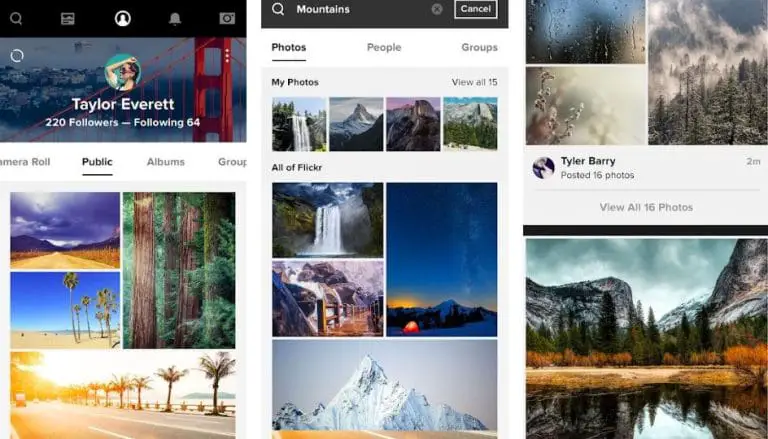The image composition consists of three distinct screenshots displaying different sections of a social media platform, with a predominant nature theme.

On the left side, the screenshot is primarily black and white. At the top, there is a black rectangular box housing several light gray tabs. On the top left is a search bar, followed by a square to its right. In the center is a circle icon with a person inside, a bell icon to the right, and a camera icon on the far top right. Below this header is a profile picture of a woman, labeled "Taylor Everett" in white text. Beneath her name, smaller text indicates "220 followers" and "following 64." Below this are four nature images: a serene forest, two desert landscapes, and a lone highway, each contributing to the natural theme.

The central screenshot exhibits a similar layout with a dark gray search bar at the top containing the phrase "mountains" in white text. The main section features a series of nature photographs, including an expansive shot of a dark blue sky, a cascading waterfall, a picturesque bridge, and a snow-capped mountain.

On the right side, the final screenshot continues the nature motif with more images. The top images showcase a rain-speckled window and a wooded landscape blanketed in snow, followed by a close-up of a flower. The bottom image captures a set of mountains under a gloomy sky, with a reflective lake below that mirrors dark trees and an orange-beige foreground.